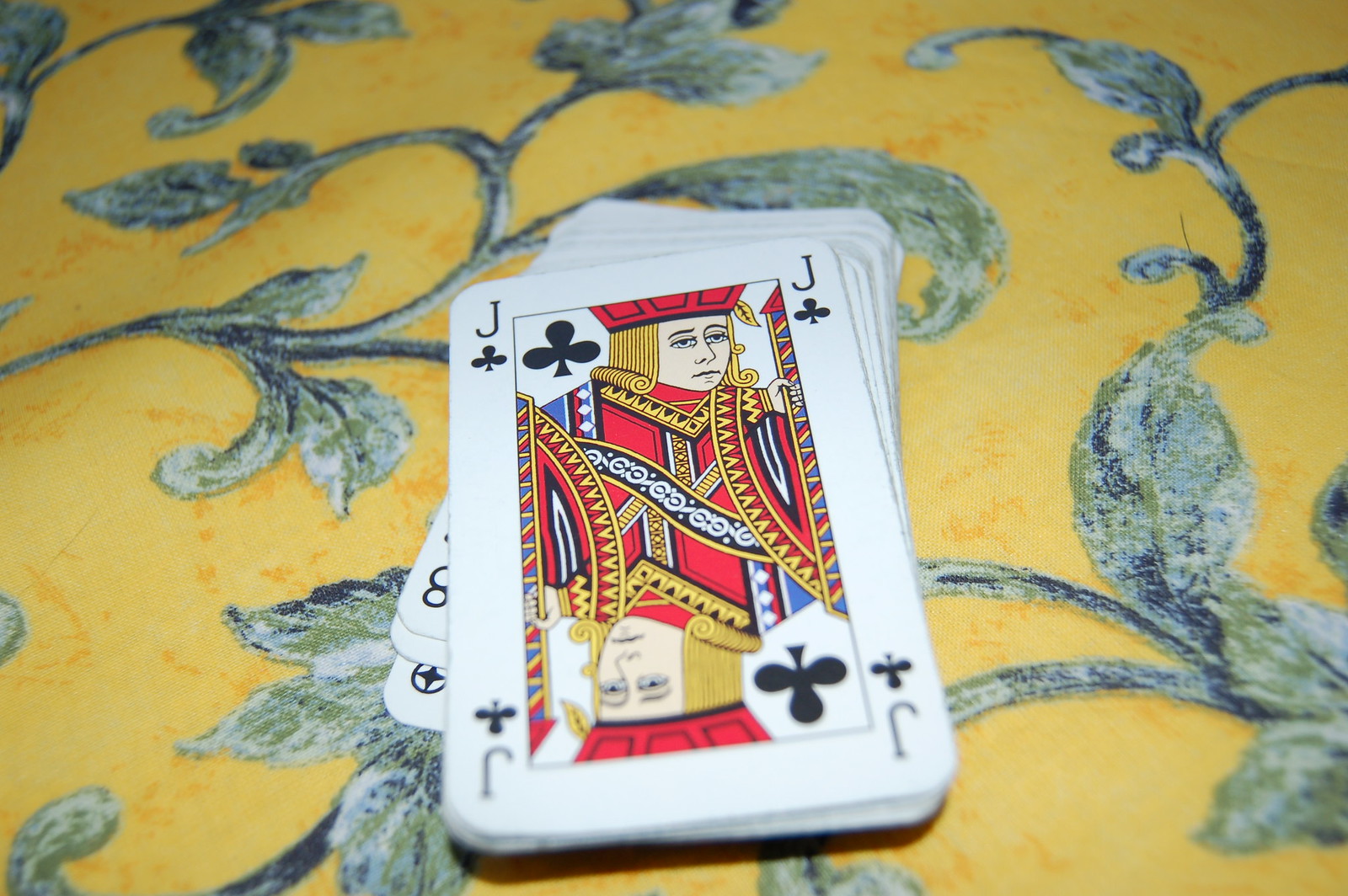This horizontal image showcases a close-up of a slightly skewed deck of playing cards placed on a richly textured yellow fabric. The background fabric exhibits a deeper canary yellow hue, adorned with splatters of darker yellow speckles and lines, interspersed with embroidered leaves in shades of green and blue. Central to the image, the deck of cards is positioned vertically, rotated slightly counterclockwise to an approximate 11:30 orientation. The bottom three cards of the deck, partially revealed and upside down, include an eight that is slightly obscured. Dominating the top of the stack is the two-eyed Jack of Clubs, drawing focus with its upper half in sharp clarity while the remainder of the image retains a soft blur.